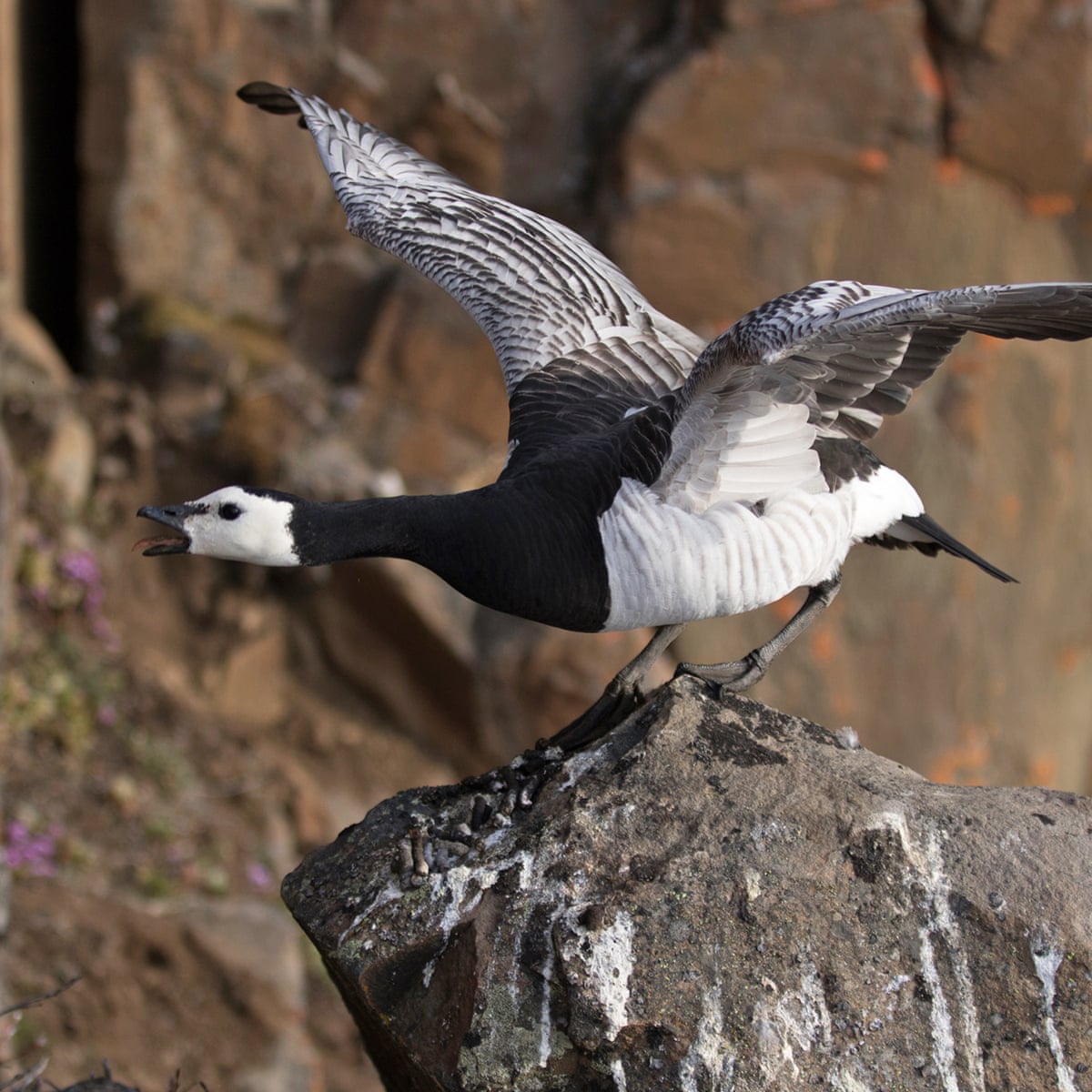In this striking photograph, a dynamic bird, possibly a goose, is perched on a substantial rock that is heavily marked with the droppings of many previous avian visitors. The scene suggests a cliff or canyon backdrop, with a blurred rock face and hints of purple flowers in the background. The bird itself is a dramatic sight with its head down, beak open, and wings spread wide as if it is squawking or poised for flight. The bird's head and breast are white, while its neck, beak, and chest are solid black. Its wings display a mix of white, black, and brown feathers, and it appears to have black feet. Adding to the intensity, its tongue is visible, further emphasizing the bird's assertive and lively posture.